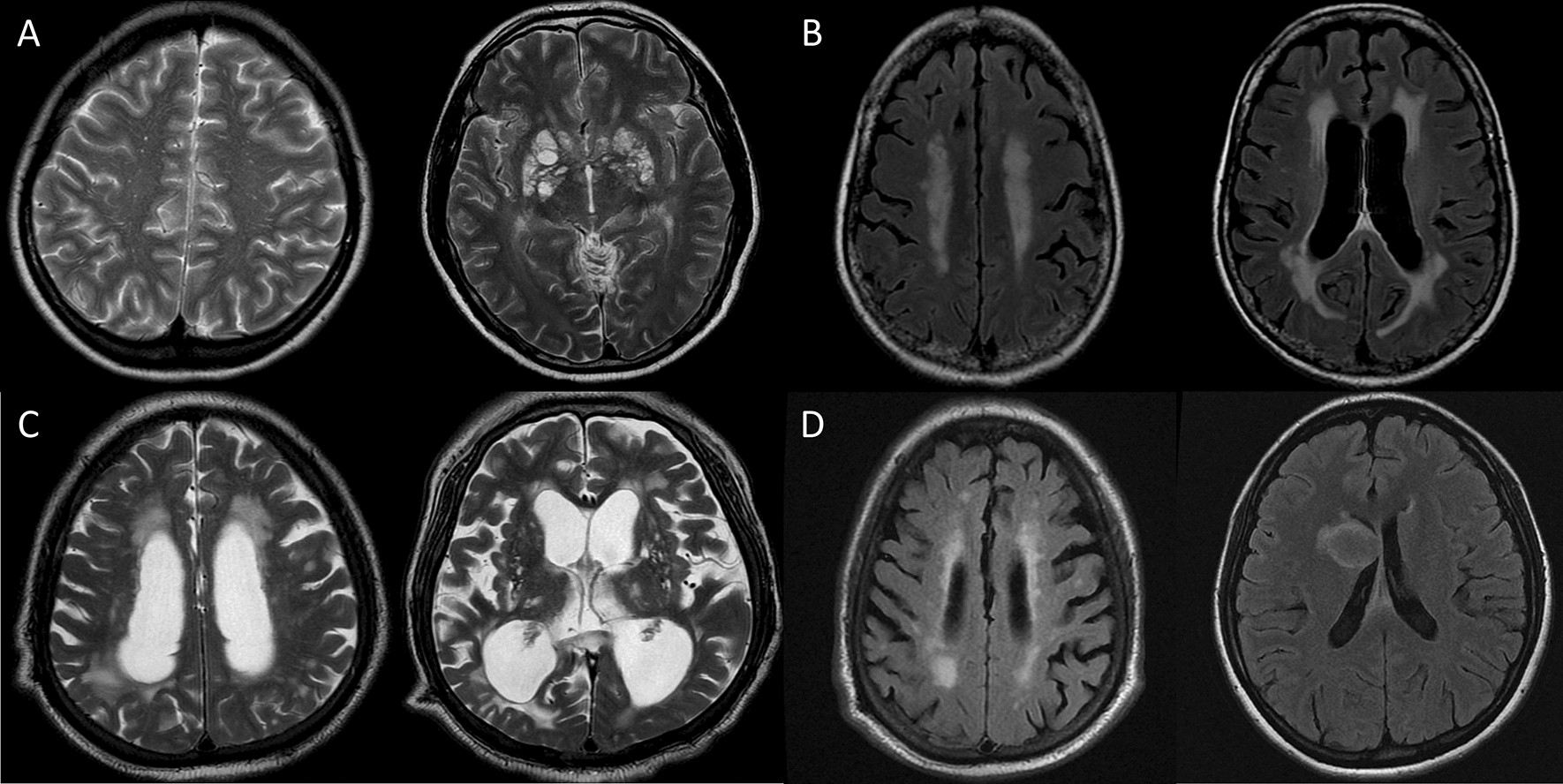This image is a comprehensive scan showcasing multiple cross-sections of what appears to be MRI scans of human brains. There are eight scans in total, categorized into four groups labeled A, B, C, and D, with each group containing two scans. The background is black, which contrasts sharply with the white and gray tones of the brain scans, highlighting various brain structures and details.

Group A appears to exhibit the frontal sections of the brain, showing bright white lines indicative of the brain’s crevices and the surrounding skull. Group B illustrates sections that seem to explore deeper into the brain, revealing structural elements like the corpus callosum with notable gray and some black regions that delineate the brain's folds and internal features. Group C comprises scans that are visually brighter, with pronounced white areas around the brain folds, suggesting even deeper sections. Group D shows the back or bottom parts of the brain, characterized by distinct but somewhat less bright areas compared to previous groups, with black lines highlighting significant structural details.

In each scan, the brain's variation in size and structure is evident, emphasizing different anatomical and possibly pathological features. The sophisticated detailing provided by this imagery suggests these scans could be instrumental in medical diagnostics or neurological studies.